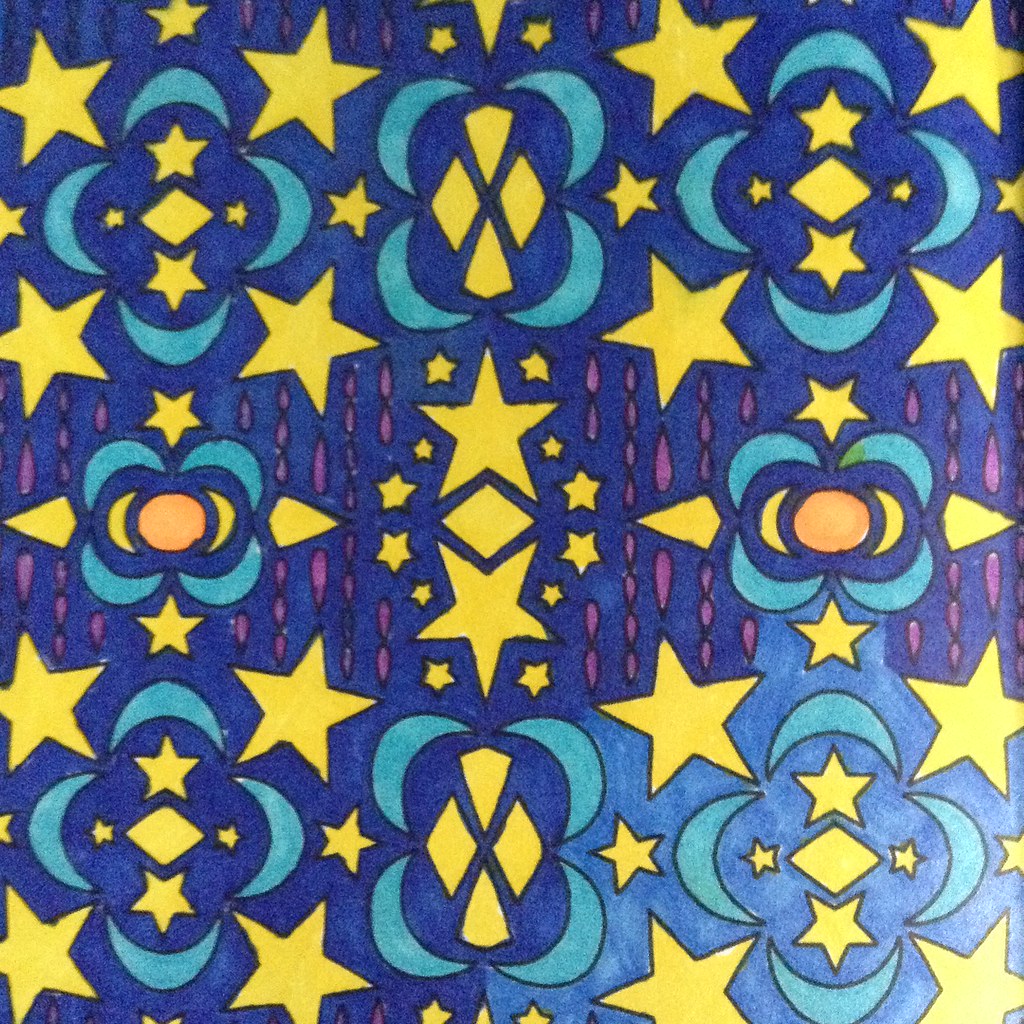This image showcases a vivid, colorful drawing or possibly a piece of fabric. The primary background color is blue, ranging from sky blue in the bottom right to navy blue elsewhere. The design features a rich collection of decorative figures and shapes, primarily in shades of blue, yellow, purple, orange, and black. Prominent throughout are numerous yellow five-point stars, each outlined in black, arranged in columns. Interspersed among these stars are various other patterns, including baby blue crescent shapes with yellow diamonds or stars inside, orange sun-like shapes, and purple raindrop-like figures. The composition is reminiscent of a mosaic, divided into three distinct sections. The first section displays a combination of stars and moon-like features, the second section features star clusters with adjacent four-part moon elements, and the third section has irregular shapes, maintaining a cohesive theme of celestial and geometric forms. The intricate design also includes elements reminiscent of Arab designs, such as clover-like shapes, enhancing the overall decorative pattern.